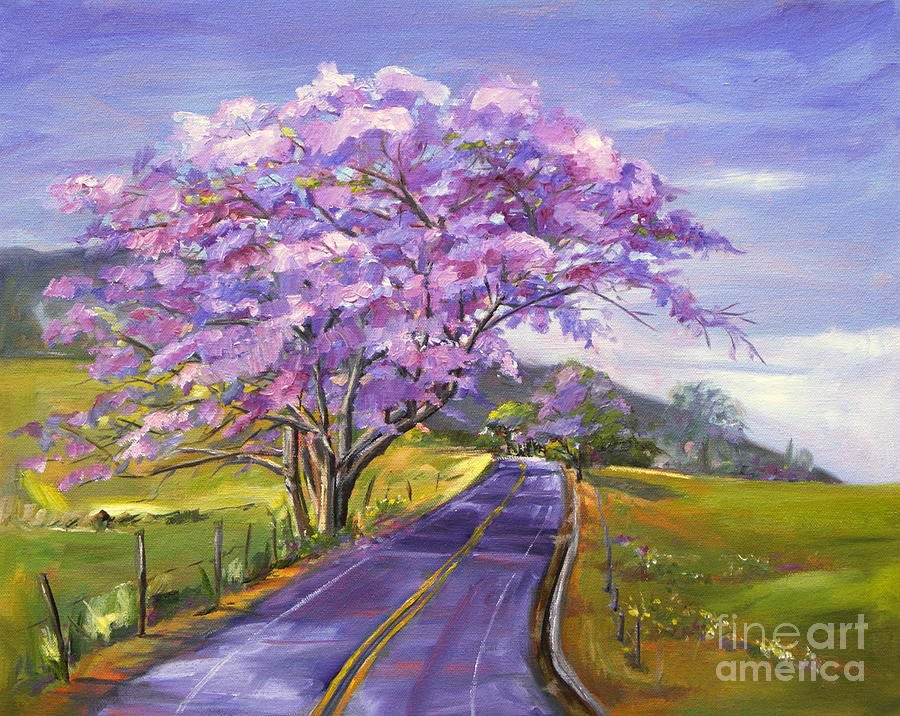The painting captures a serene country scene from the perspective of a paved road with double yellow lines extending through the center. On either side of the road lie expansive grassy fields dotted with small flowers in shades of yellow and purple. A weathered wooden fence with posts and wires runs along the edge of the road. Dominating the composition on the left side is a majestic tree with branches extending over the road. This tree features a striking blend of whitish and purplish leaves, and its vibrant purple hue casts a mesmerizing reflection onto the road beneath it. Behind the tree, the landscape gently slopes into a large hill painted in a darker green. The sky above transitions from a deep blue at the top to a lighter, almost white shade as it meets the horizon, interspersed with wisps of white clouds and a subtle purple tinge.